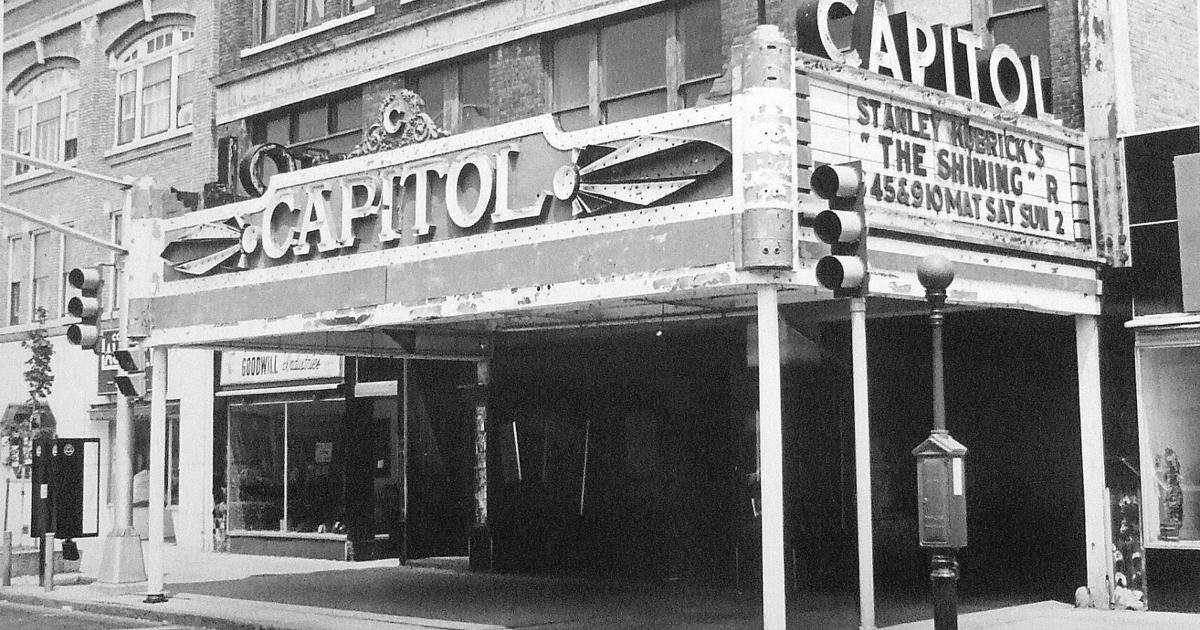This detailed black-and-white photograph captures an old movie theater called "The Capitol," situated on what appears to be a corner building with apartments above it. The marquee prominently displays "Stanley Kubrick's The Shining," rated R, with showtimes listed as 6:45 and 9:10, and a matinee on Saturday and Sunday at 2. The theater's name, "Capitol," is spelled out in large, 3D letters on both the front and side of the awning, supported by columns. The scene includes traffic lights on either side of the theater, suggesting an intersection. The architecture has an Art Deco flair, with decorative elements enhancing the signage. Adjacent to the theater, a Goodwill store can be seen, indicating the theater is part of a small-town streetscape.